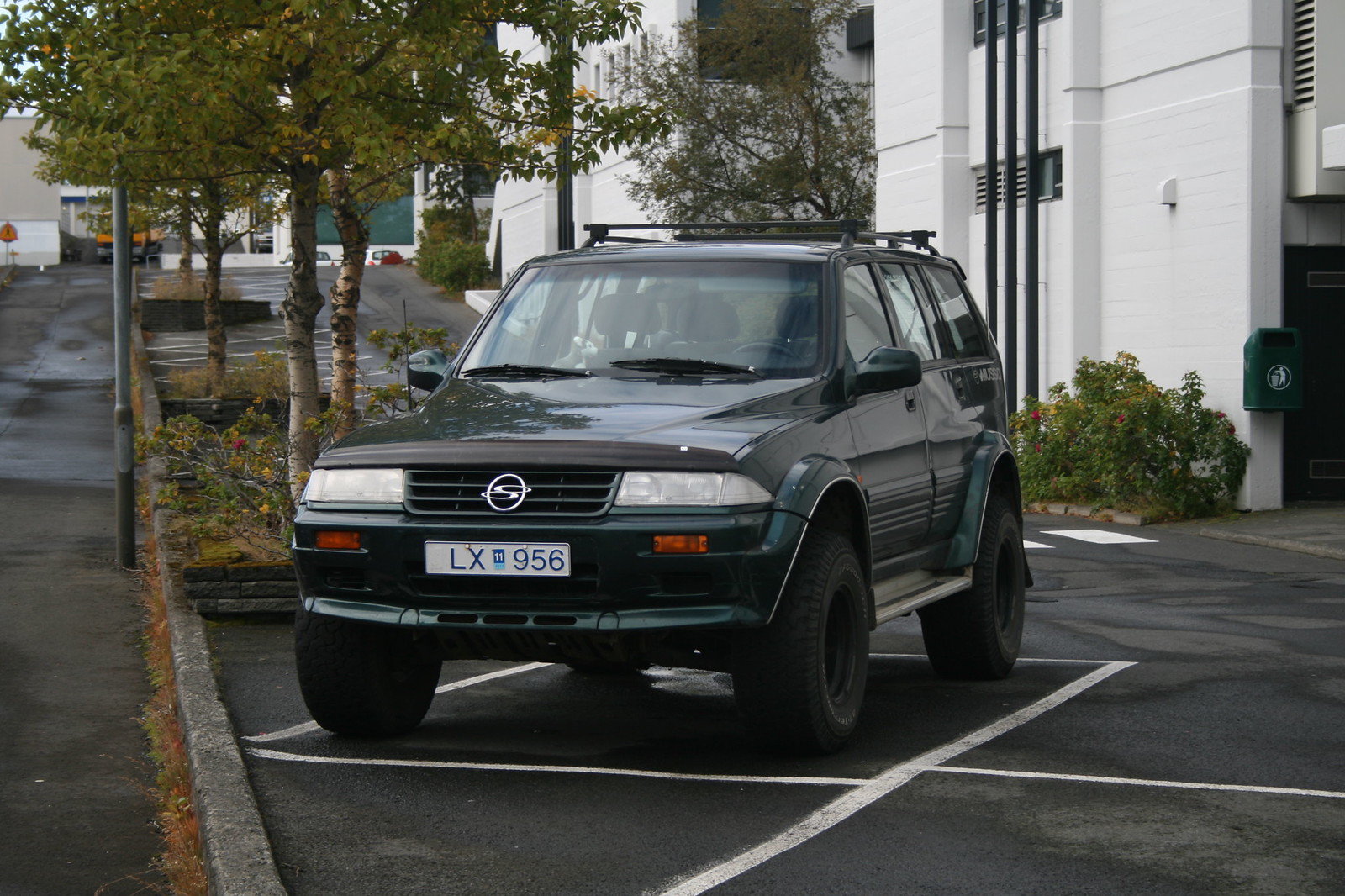The photograph depicts a dark green SUV, resembling a small jeep, positioned at a slight angle facing mostly forward and slightly to the left. It's situated in a marked parking spot adjacent to a curb, with a street and trees visible on the left. The vehicle has four doors and features a black roof rack and an indistinct symbol resembling an 'S' on the front grill. The license plate reads "LX956" with blue text on a white background. A white building, visible in the upper right, extends down the parking area and includes a door on the right side of the image. The parking area shows an uphill inclination to the left, leading to additional parking spaces lined with trees in wooden borders. In the distant background, an orange vehicle and a triangular orange sign are visible, along with two more white vehicles parked further up the hill. The scenery includes a mix of concrete surfaces, trees, bushes, and segments of streets and buildings.